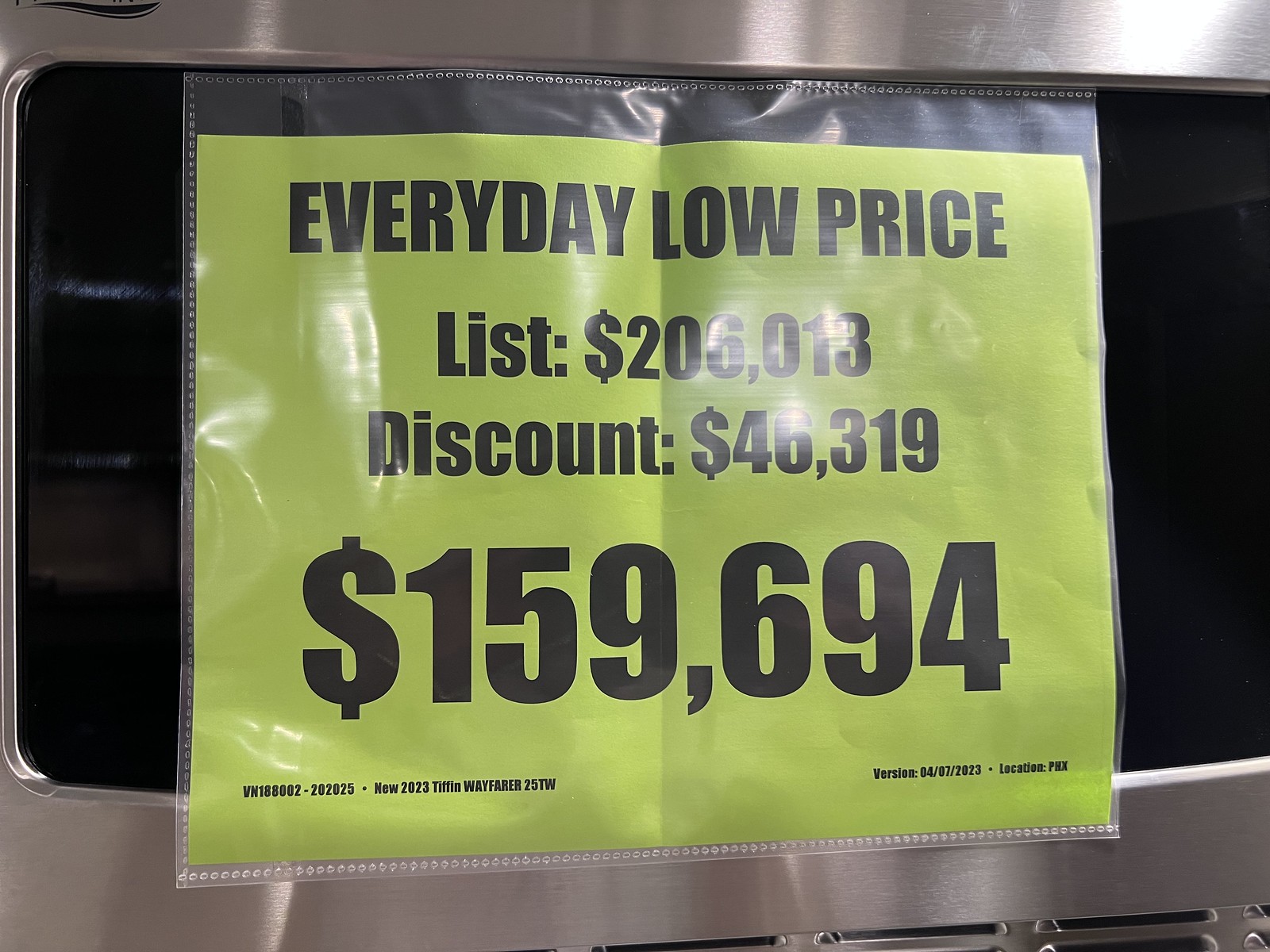The image is a close-up color photograph showing a price tag on what appears to be a high-end appliance, most likely an oven. The appliance features a black rectangular window set against a stainless steel background with grating visible near the bottom. The laminated green price tag is affixed to the black window, containing several price details in bold black print. The tag prominently displays the text "Everyday Low Price" followed by "List: $206,013" and "Discount: $46,319." The final price is stated as "$159,694." Additionally, the bottom left corner of the tag includes a detailed product identification: "VN188002-202025, New 2023 TIFFIN Wayfarer 25TW," while the bottom right corner notes "Version 04-07-2023, Location PHX." The overall appearance of the tag with its fluorescent yellow color and organized information draws immediate attention to the pricing details.